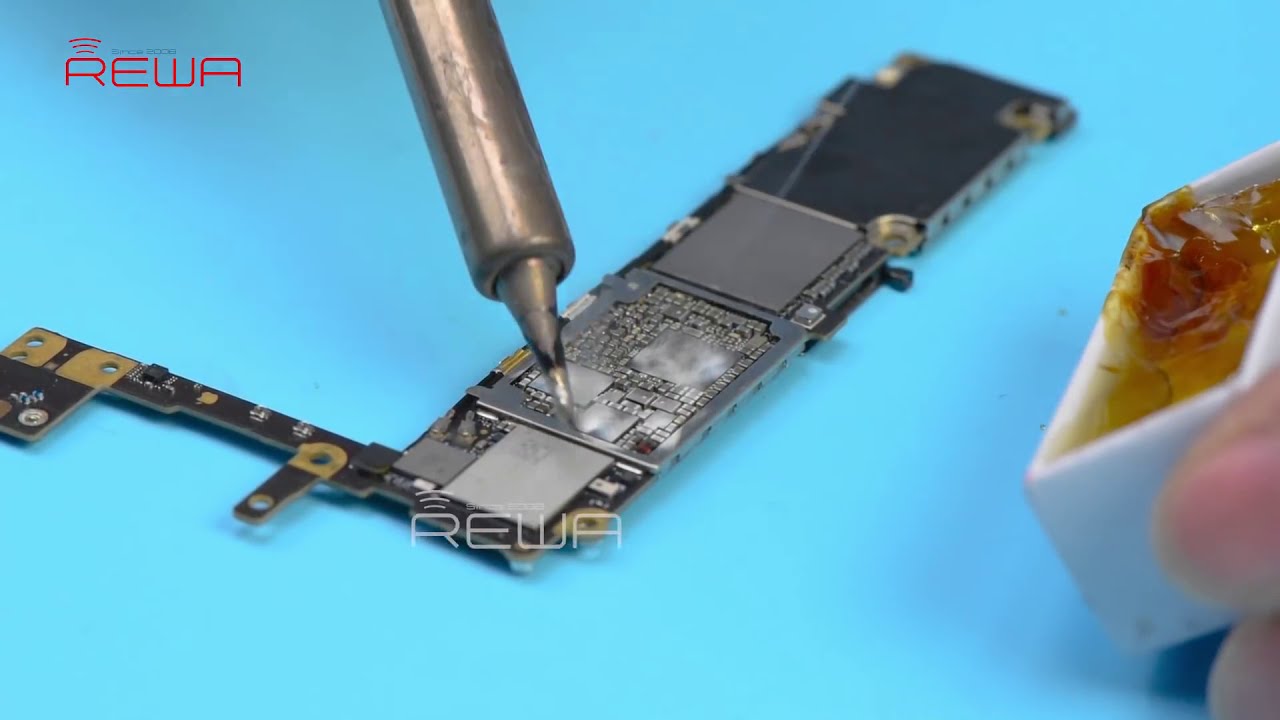The image features a detailed close-up of an electronic circuit board resting on a solid baby blue background. Prominently written in bold red capital letters in the upper left-hand corner is "R-E-W-A," with additional tiny blue lettering and a Wi-Fi symbol above the "R". The circuit board, primarily rectangular, starts from the middle left and extends upwards and to the right, with its intricate components clearly visible. A precise metal tool resembling a soldering iron gently touches the tiny parts of the circuit board, suggesting a delicate operation. To the right, part of a person's fingers emerge from the edge of the frame, holding a small white rectangular container filled with a golden, gel-like substance. The fingers are visible only partially, showing just the tips and fingernails.